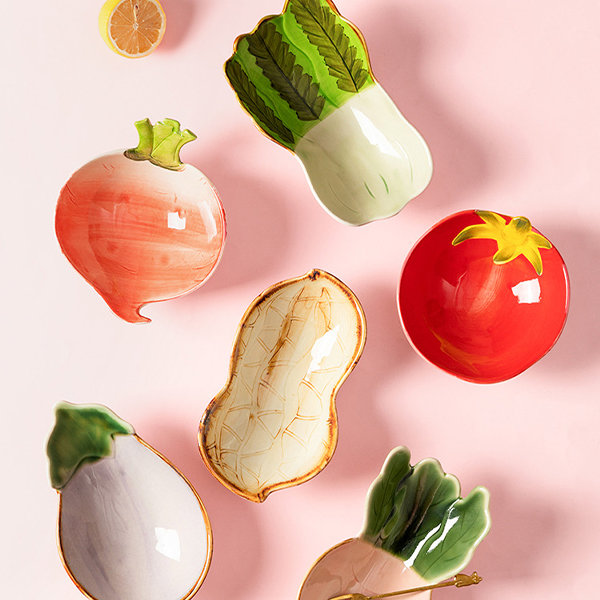This image portrays a set of intricate ceramic ornaments shaped like various vegetables and fruits. Positioned against a pink background and casting distinct shadows, these porcelain replicas exhibit a notable luster that confirms their artificial nature. The top left features a small orange or grapefruit, followed by a tomato sitting prominently below. Adjacent to the tomato is a head of cabbage or romaine lettuce. Moving downward, there is a radish and to its right, an eggplant. Further below is a peanut-like shape, and at the very bottom, there is a daikon or possibly a rutabaga. These beautifully crafted pieces are not only visually accurate but also versatile, as their hollow insides suggest they can be used to hold small items like nuts or candies. This collection captures the delicate artistry and realism of ceramic craftsmanship.